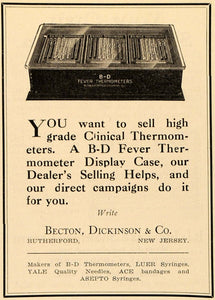This is a vintage newspaper advertisement with a tan background and a black line border that frames the entire page. At the top, there is an image of a black, rectangular display case with a clear glass top, designed to showcase high-grade clinical thermometers. The advertisement prominently features bold black font that reads: "You want to sell high-grade clinical thermometers," followed by, "A B-D fever thermometer display case - our dealer selling helps and our direct campaigns do it for you." Beneath this, in a lighter font, it states: "Wright, Becton, Dickinson & Company, Rutherford, New Jersey." A black line separates this from the text at the bottom that lists the company's products: "Makers of BD thermometers, Luer syringes, Yale quality needles, Ace bandages, and Asepto syringes." The overall design gives off an old-fashioned and professional appearance, befitting a historical advertisement.